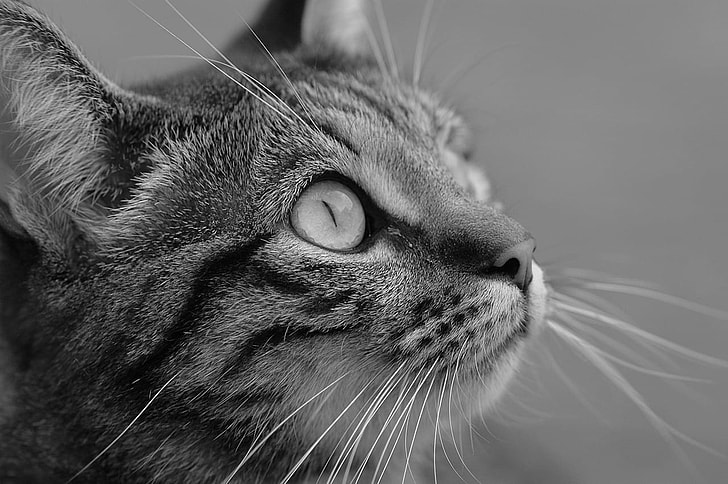This is a black and white photograph in landscape mode of a tabby cat's face, captured in a detailed, close-up profile. The cat, likely a common house cat, is peering intently at something in the upper right corner that remains out of the frame. The photograph prominently features the right side of the cat's face, showcasing its intricate tabby markings—darker stripes beside and under its eyes, as well as on the top of its head. The cat's eyes are wide open, with clear, light irises and small vertical slits for pupils, expressing a look of focused curiosity. Its nose is positioned at the front right of the image, and the numerous white whiskers above the eyes and around the face are sharply defined. The left ear is almost fully visible with noticeable fur inside, and part of the right ear and the top of the head are also in frame. The photograph has a gray blurred background, ensuring all attention remains on the cat’s detailed and handsome face.